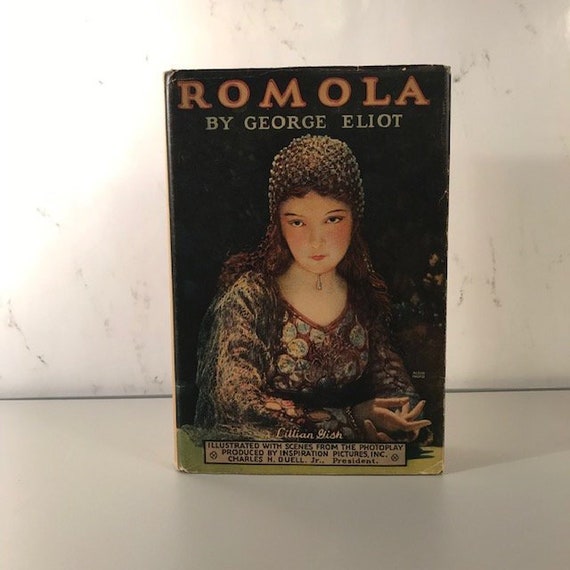The image depicts a dimly lit, color photograph of an antique book positioned against a white marble wall on a light gray surface, possibly a desk or floor. The book, titled "Romola" in orange capital letters, is authored by George Eliot and has a black background. The cover features an illustration of a woman identified as Lillian Gish, a notable actress. She has long, curly brown hair adorned with a net-like, bejeweled head covering. The illustration shows Gish with rosy cheeks, small lips, and brown eyes, wearing a velvet-like dress with a floral print, gauzy sleeves, and a choker necklace with a pendant. Her hands are crossed, palms up, resting on a table. At the bottom, a box indicates that the book is illustrated with scenes from a photoplay produced by Inspiration Pictures Incorporated. The hardcover book has a paper slipcover, further indicating its antique nature.